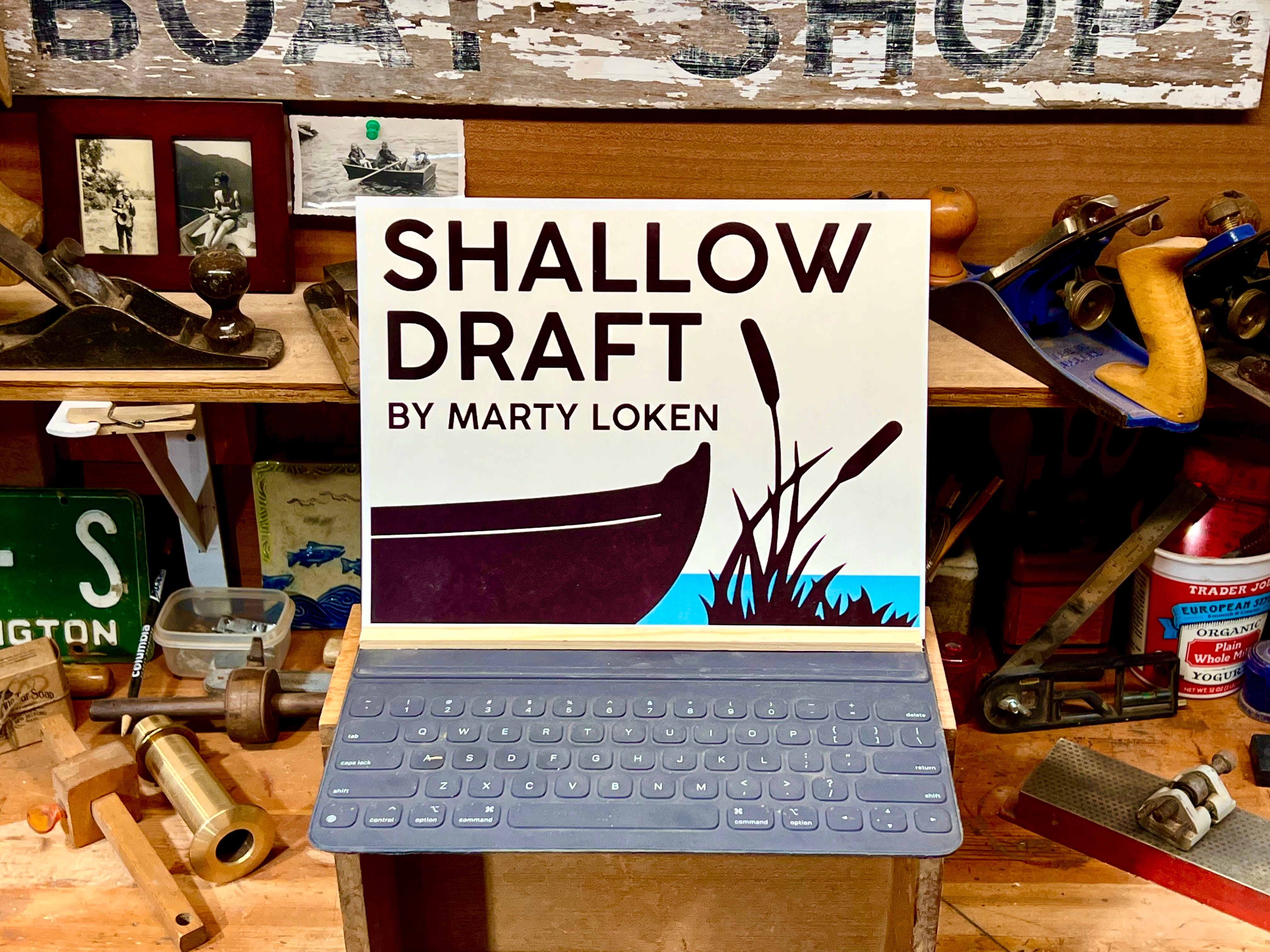In the image, we see a bustling woodshop filled with various tools and items. The central focus is a black keyboard on which sits a sign that reads "SHALLOW DRAFT by Marty Loken," featuring an illustration of a boat and some cattails. The background reveals wooden shelves holding an assortment of metal and wood tools, including lathes, files, sanders, and clamps. A laptop is also prominently displayed, echoing the same "Shallow Draft by Marty Loken" title on its screen. In the top left corner, two black-and-white photographs in deep mahogany frames can be seen. Additionally, a shabby, white-painted wooden sign with chipping paint and the words "BOAT SHOP" in black text is mounted on the wall. The workspace also includes a license plate and an empty Trader Joe's yogurt container repurposed to hold more tools, all contributing to the cluttered yet industrious atmosphere of the woodshop.